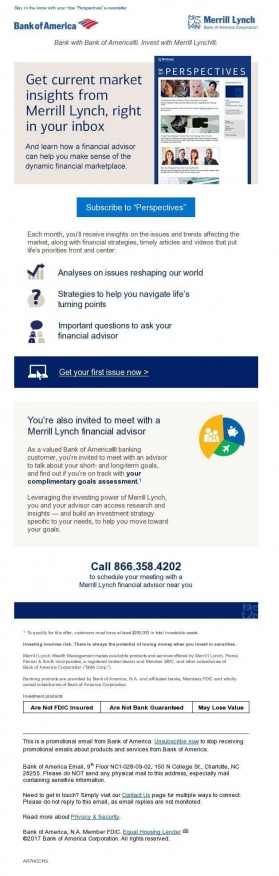**Descriptive Caption:**

This image presents a detailed and informational promotional ad for Merrill Lynch, a subsidiary of Bank of America. The central theme is to encourage users to subscribe to Merrill Lynch's market insights and financial advice newsletters. 

At the top left of the image, there's a small hyperlink, followed by the Bank of America logo. To its right, the Merrill Lynch icon can be seen, with the text "Merrill Lynch" beside it. Beneath this, the text "Bank of America Invest in Merrill Lynch" is displayed prominently.

The main section of the ad, which has a gray overlay with dark blue text, features the following call to action: "Get current market insights from Merrill Lynch, right in your inbox." Below this in white text against a dark blue background, the word "Perspectives" is written, and it is followed by various images. The ad elaborates with: "Learn how a financial advisor can help you make sense of the dynamic financial marketplace," suggesting the value of subscribing.

To subscribe, users are directed to click a light blue hyperlink box labeled "Subscribe to Perspectives." Further white text elaborates: "Each month you will receive insights on the issues and trends affecting the market, along with financial strategies, articles, and videos that put your priorities front and center."

In the lower section, dark blue text highlights three main focuses:
1. "Analysis on issues shaping our world."
2. "Strategies to help you navigate life's turning points."
3. "Important questions to ask your financial advisor."

Finally, there is a call-to-action button encouraging users to get started. The image concludes with two more text blocks containing approximately 200-300 words each, providing additional details and information.